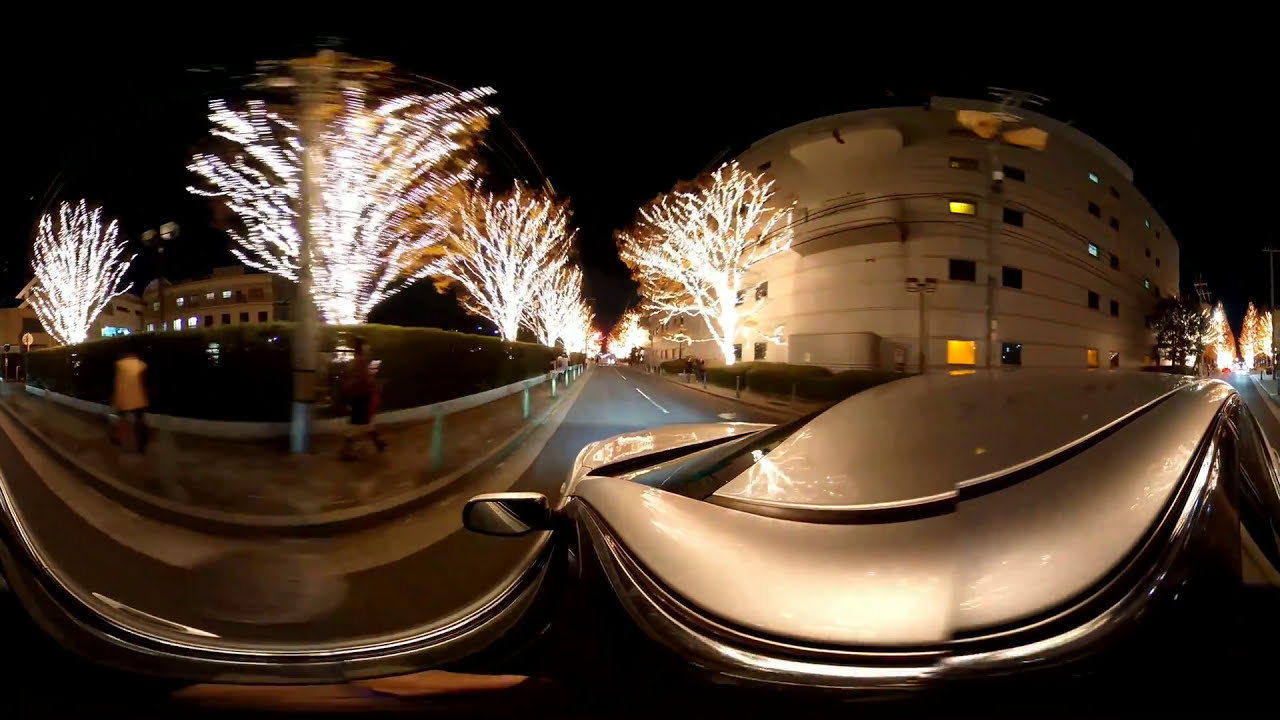The photograph, taken at nighttime through a car windscreen, presents a slightly distorted view of an urban scene. In the foreground, a silver vehicle with its roof and side view mirror visible is positioned towards the bottom center. The road ahead is flanked by guardrails and a walking path where two blurred figures, one in a red coat and the other in a yellow coat, are seen strolling on the sidewalk to the left. Both sides of the road are lined with lit-up trees, their lights casting a warm glow against the dark night sky, which takes up the top quarter of the image. 

To the right, a large, rounded building with numerous windows is partially obscured by a hedgerow. Additionally, more illuminated trees extend along a side road to the far right, adding depth to the scene. The photograph captures the contrasting elements of bright lights and deep shadows, vividly conveying the serene yet bustling ambiance of the nighttime urban landscape. No text is present in the image.